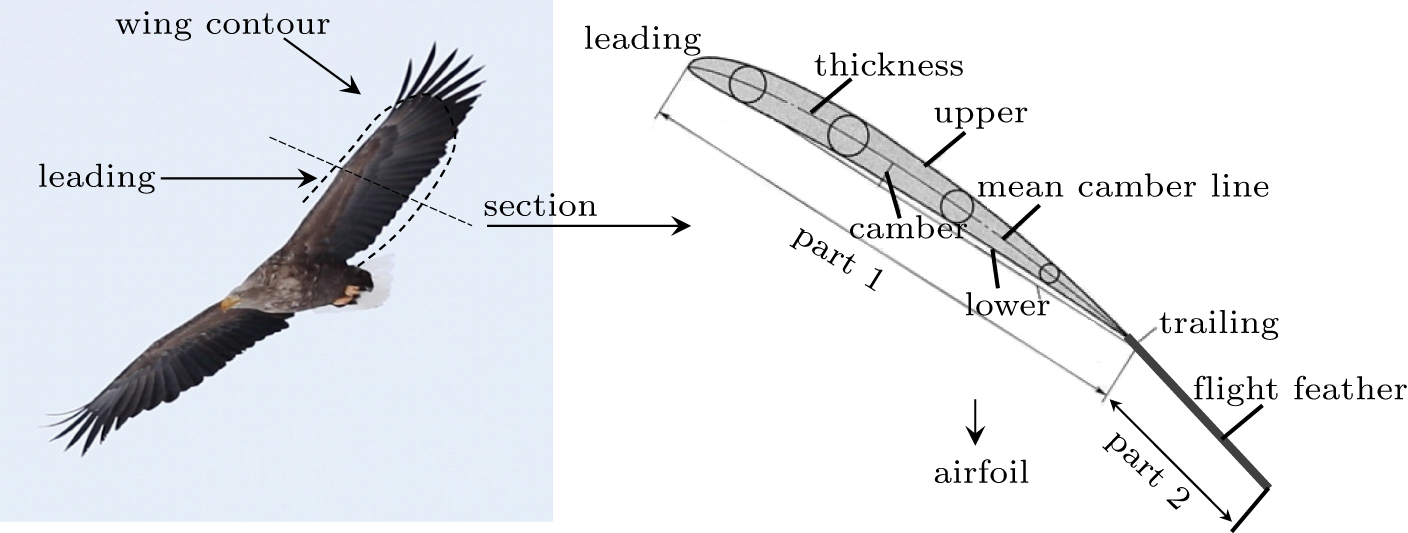The image is a detailed, rectangular illustration divided into two sections, each measuring approximately five inches wide and two inches high. On the left side, within a square light-blue background adorned with dotted lines, there is a dark-colored bird, possibly an eagle, in mid-flight with its wings outstretched diagonally—the right wing pointing to the upper right corner and the left wing to the lower left corner. This bird image features various labeled parts such as "wing contour," "leading," and "section," which is indicated by arrows and circles directing attention to specific features of the wing.

The right side of the image showcases a detailed, black-and-white diagram of a bird's wing, highlighting its anatomical and aerodynamic aspects. This diagram is partitioned into "Part 1" at the top and "Part 2" at the bottom, with numerous labels detailing various components: "leading," "thickness," "upper," "camber," "mean camber line," "lower," "airfoil," "trailing," and "flight feather." Each section and term is connected by arrows, making it an informative illustration of wing structure and function.